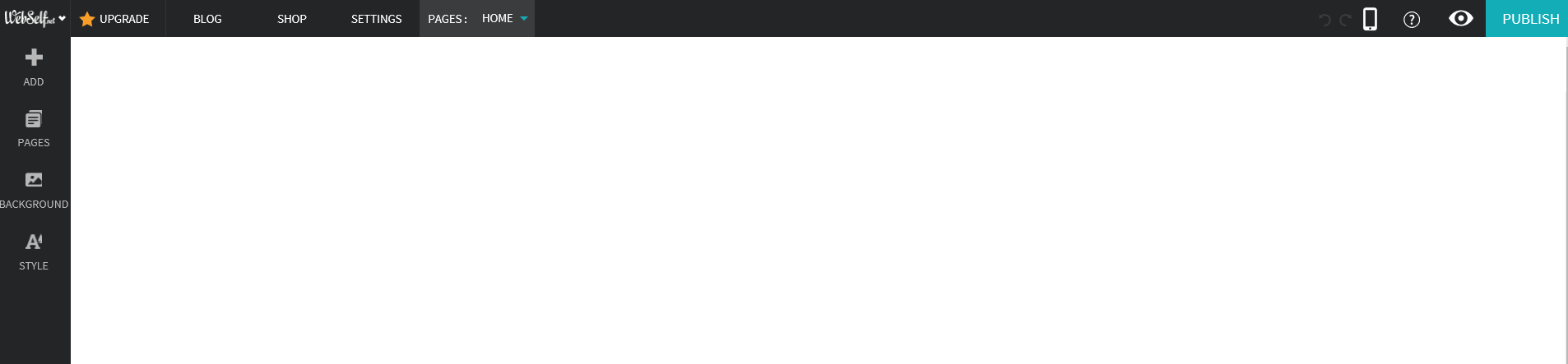This image appears to be a screenshot of a user interface, likely from a design or web layout application. The main part of the image is predominantly white, comprising about 95% of the total view. At the very top, there is a horizontal menu bar with items listed in a small, unreadable logo followed by an orange star icon. To the right of the logo, menu options labeled "Upgrade," "Blog," "Shop," "Settings," "Pages," and "Home" are displayed in grey text.

A thinner vertical menu bar runs along the left side of the image. This bar contains several icons and labels from top to bottom: a plus sign alongside the word "Add," a pair of stacked rectangles presumably labeled as "Pages," an image icon resembling a photo with a dot and a mountain, labeled "Background," and a capital 'A' with the word "Style" next to it.

On the right side of the top horizontal menu, adjacent to the text options, there are additional icons and elements. These include a phone icon, an eye-shaped icon, and a prominent blue button labeled "Publish." On the extreme right edge of the image is a nearly invisible, one-pixel grey line.

The logo at the top is written in a script or handwriting style and is approximately eight to ten pixels tall, making it unreadable and thus not identifiable.

Overall, the interface suggests the image is from a design tool or webpage layout application, aimed at facilitating the creation or management of digital content.